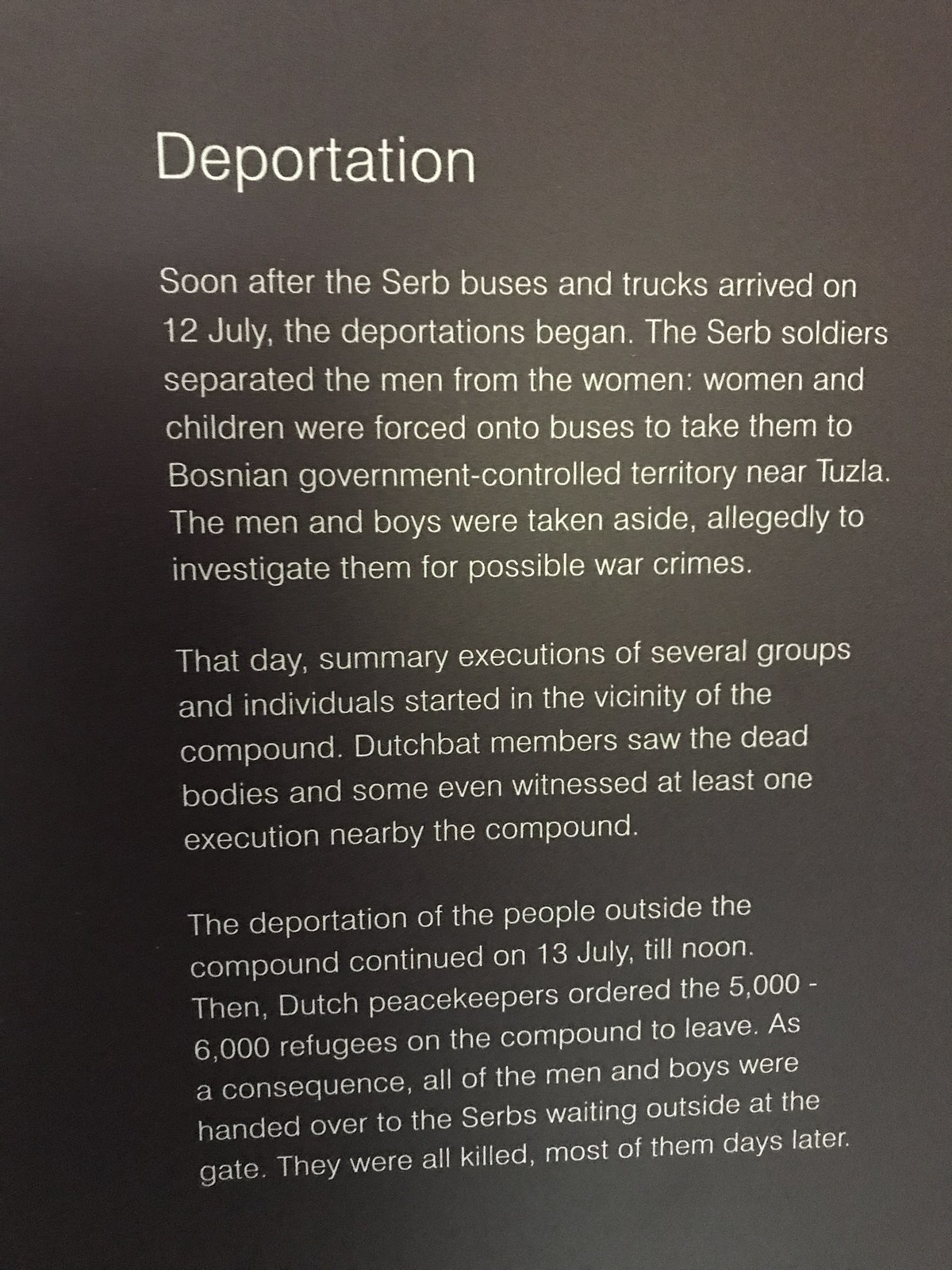The image appears to be a slightly slanted photograph of a dark gray or black page, possibly from a book or a poster, with clean white text prominently detailing a historical account of deportation. At the top, the word "Deportation" is written in large white letters. Below this title are three detailed paragraphs. 

The first paragraph states: "Soon after the Serb buses and trucks arrived on 12 July, the deportations began. The Serb soldiers separated the men from the women. Women and children were forced onto buses to take them to Bosnian government-controlled territory near Tuzla. The men and boys were taken aside, allegedly to investigate them for possible war crimes."

The second paragraph describes: "That day, summary executions of several groups and individuals started in the vicinity of the compound. Dutch peacekeepers witnessed the dead bodies, and some even saw at least one execution nearby the compound."

The third paragraph explains: "The deportation of the people outside the compound continued on 13 July until noon. Then Dutch peacekeepers ordered the 5,000 to 6,000 refugees inside the compound to leave. All the men and boys were handed over to the Serbs waiting outside at the gate, where they were all killed, most of them days later."

The overall image captures a grim narrative of the events surrounding the deportations, emphasizing the tragic fate of the men and boys, and the witnessed atrocities during the ordeal.